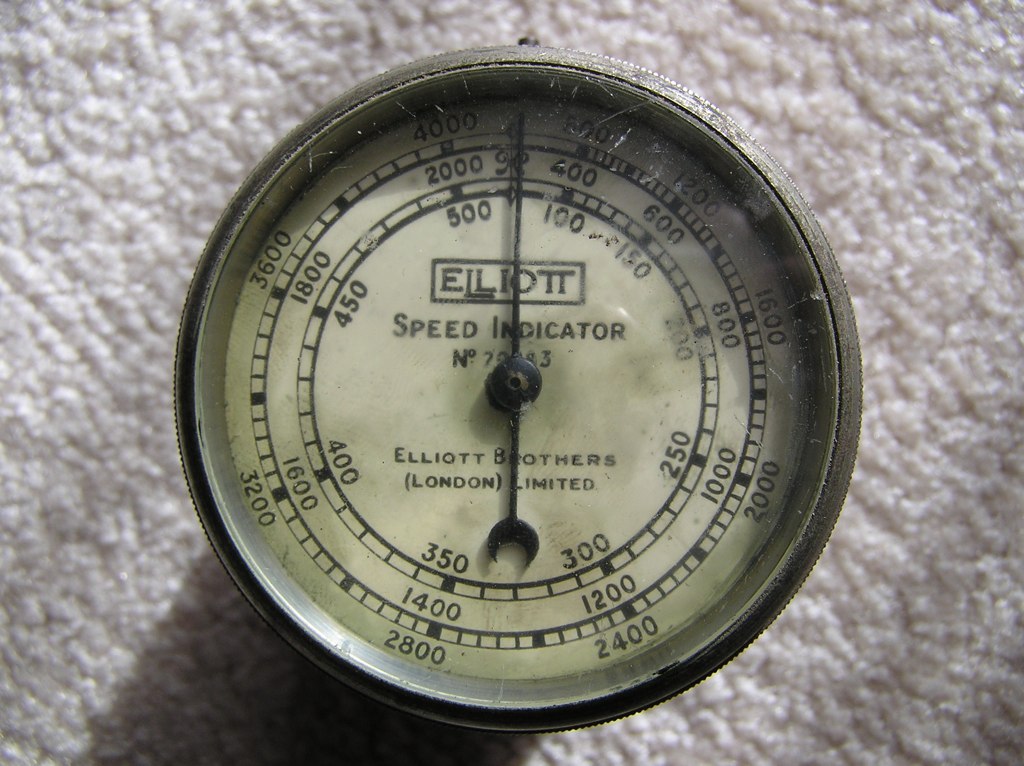The image depicts a vintage speed indicator gauge encased in a robust metal housing. The top of the gauge features a dark-colored button or knob, suggesting a possible calibration or reset function. The face of the gauge is covered by a flat, glass or plastic surface revealing a white dial beneath. The central region of the dial bears the word "Elliott" in bold black letters, surrounded by a black outline. Below this, the gauge is marked "Speed Indicator" with a partially obscured number, presumably indicating the model.

Further down, the text reads "Elliott Brothers London Limited" with "London" specified in parentheses. The numerals encircle the gauge face in multiple tiers: the outermost numbers, though partially shaded, range from 1,200 to 4,000 at intervals of four hundred units. Inside this, a black and white marked ring displays incremental tick marks paired with larger frequencies labeled 2,000, 4,000, 6,000, 8,000, 1,000, 1,200, 1,400, 1,600. The innermost tier of the gauge displays numbers in smaller increments of fifty, ranging from 500 to 400.

This intricate and clearly labeled setup indicates that the gauge measures speed, most likely engine speed or RPM, produced by Elliott Brothers in London.